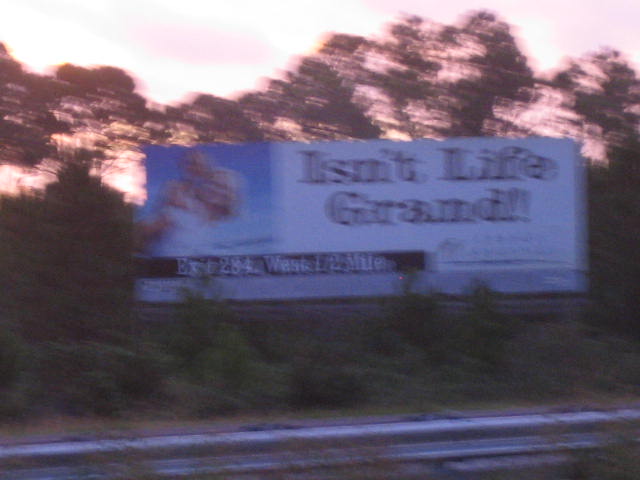A blurry photograph captured from a moving vehicle showcases a large billboard on the side of a highway. The scene is framed by lush bushes and shrubbery with tall trees in the background, suggesting either sunrise or sunset from the warm, diffused lighting. In front of the billboard, a metal barrier stretches along the road, partially obscured by weeds or small bushes.

The billboard itself features a partially discernible image of a smiling blonde person in a white t-shirt, possibly carrying a child or another person on their back, set against a bright blue sky. Adjacent to this image is a white section with bold black text that reads "Isn't life grand!" An additional black stripe beneath the main text contains the words "Exit 284 West, 1/2 mile," also in white lettering. The rest of the billboard's details are blurred beyond recognition, rendering them indecipherable.